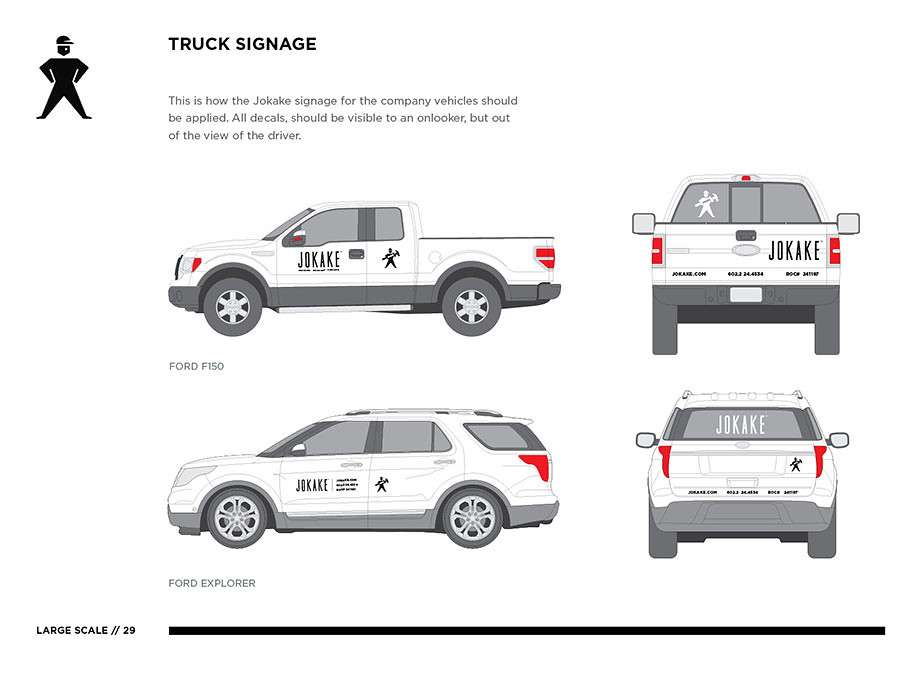The image is an instructional guide for applying Yokake signage to company vehicles, specifically depicting a Ford F-150 and a Ford Explorer. The title "Truck Signage" is prominently displayed at the top, along with an illustration of a worker. The guide outlines the proper placement of decals so they are visible to an onlooker but do not obstruct the driver’s view. There are four digitally rendered images of the vehicles arranged in a window pane style: two images on top showing side and rear views of the Ford F-150 and two on the bottom showing the same views for the Ford Explorer. The decals should be placed on the driver's side door, the back side door, the rear glass, and the trunk area of each vehicle. The overall color scheme includes black, white, gray, and red. This detailed illustration serves as an instructional pamphlet, emphasizing the correct application of the Yokake signage.